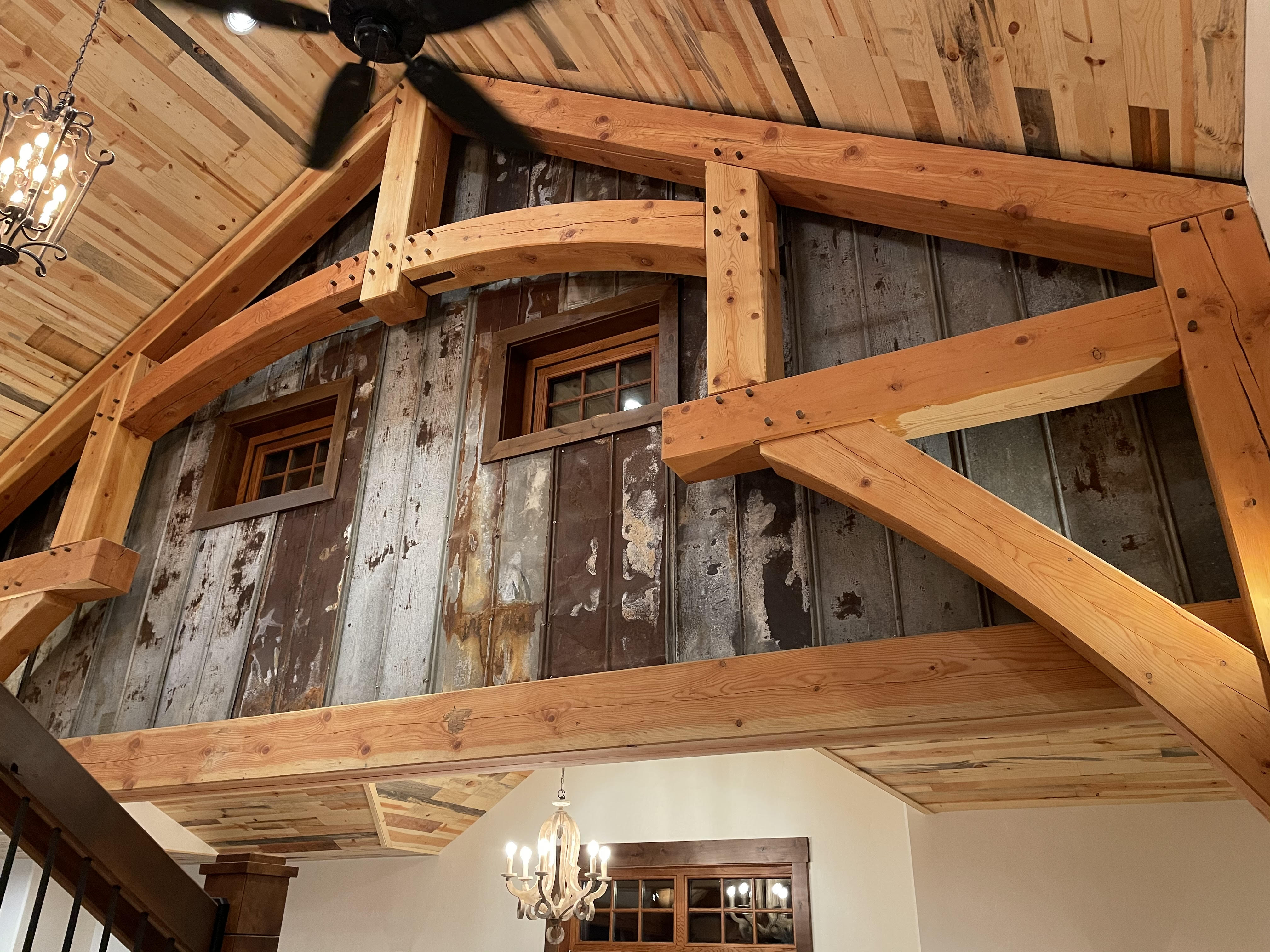The photograph captures the interior of a house with a stunning blend of aged and modern elements. Dominating the scene is a section of weathered, barn-like wood wall, evocative of a rustic exterior, juxtaposed with newer wooden scaffolding or joists that appear to support the ceiling. This striking feature is set against a remodeled room featuring plaster walls beneath the old wood, and an exquisite hardwood-like ceiling above. The ceiling is adorned with a brown, black-bladed ceiling fan located near the center, enhancing the room's vintage charm. 

Towards the top left corner, an antique-style light fixture hangs, adding to the room's classic aesthetic. Below this focal point, the lower section reveals white plaster walls harmonizing with the home's overall renovated feel. In the center of the image, gray and dark gray vertical panels accentuate the upper floor, where two small rectangular windows with brown wooden frames can be seen. These windows, possibly part of a small attic-like structure, appear to let in light through their glass panes, complementing the room's light and dark wood contrast. Additionally, the partial view of a staircase railing in the bottom left corner suggests a layered and textured architectural design, blending the historical elements with contemporary touches seamlessly.